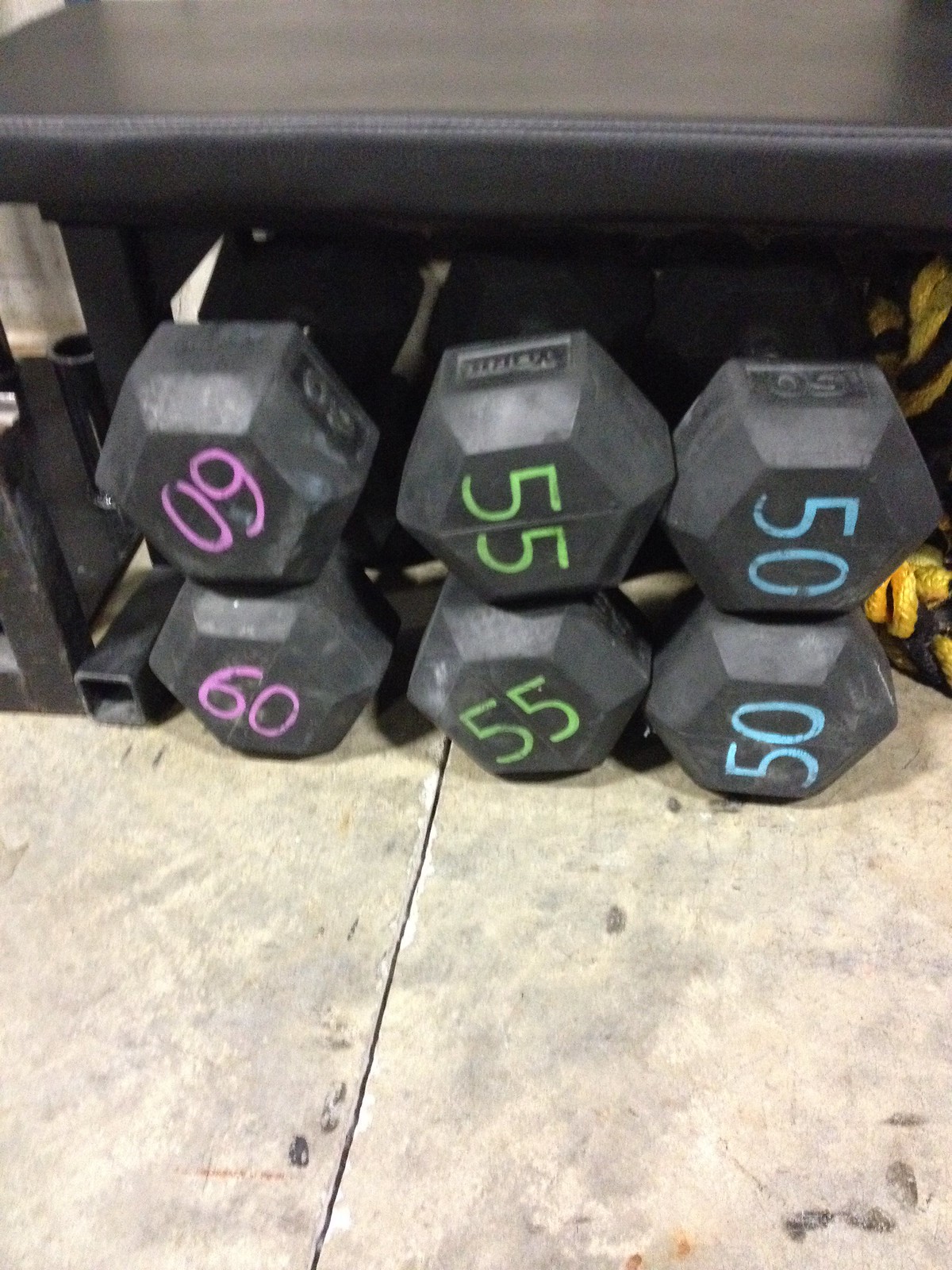In this detailed photograph, we observe six black dumbbells situated on a light gray, streaky concrete floor. The dumbbells are plastic-coated with hexagonal capping at the weighted ends. They are organized into three distinct pairs, neatly stacked one on top of the other. On the left, there are two 60-pound dumbbells marked with pink numbers. In the middle, two 55-pound dumbbells display green numbers, and on the right, two 50-pound dumbbells feature blue numbers. Above the dumbbells, there's a black leather gym bench, providing a backdrop. Some additional items, possibly a pair of gloves, in yellow and black, are slightly obscured behind the dumbbells, adding more depth and context to the gym setting.